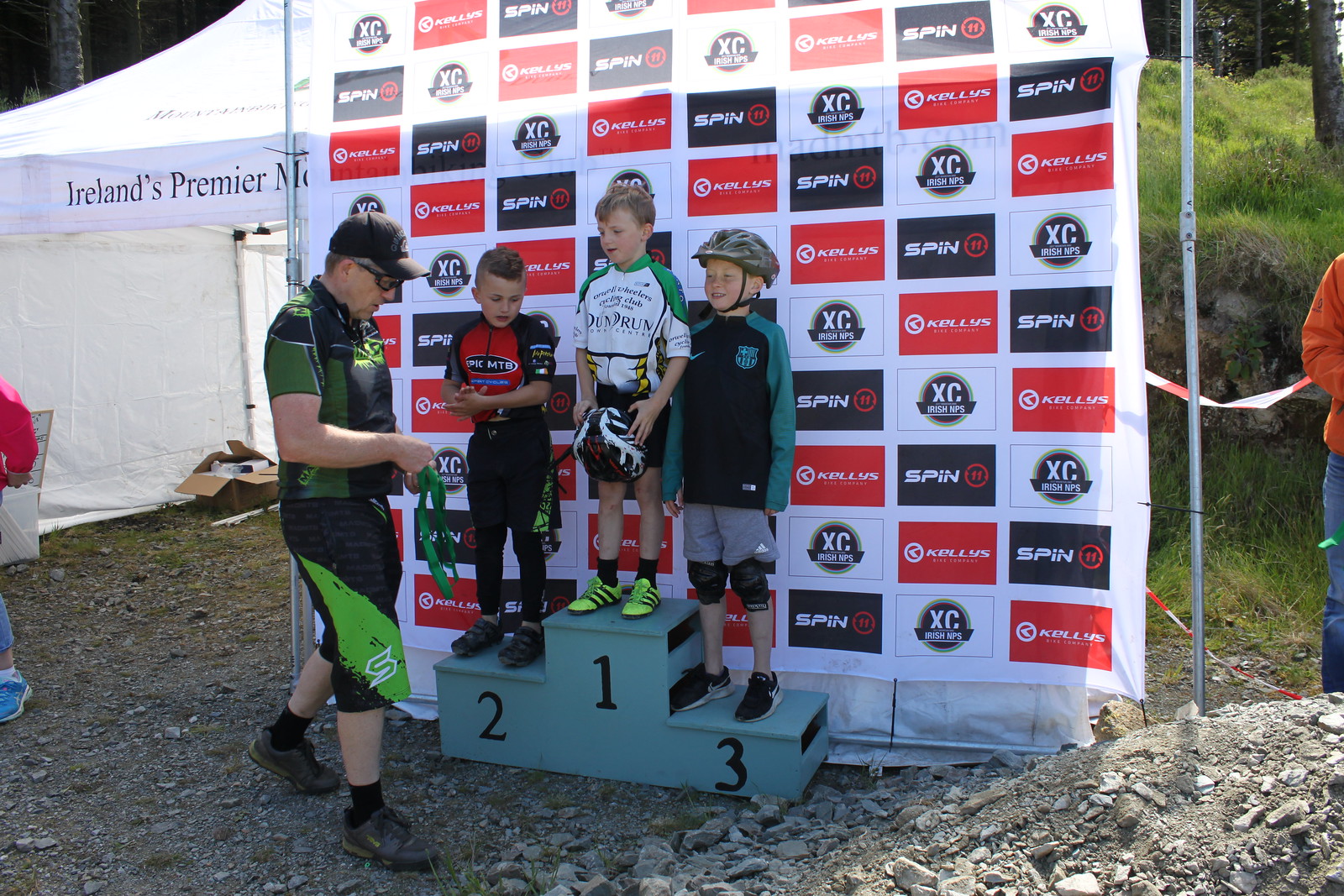The photograph captures a vivid moment of triumph at a bike race event, featuring three young boys standing proudly on a gray award podium placed on a rocky ground. Each section of the podium is labeled with large black numbers: 1 in the middle, 2 on the left, and 3 on the right, with the central platform being the highest. The boys are dressed distinctively: the center boy, dressed in a white shirt, holds a helmet in front of him; the boy to the left, sporting a red shirt and black pants, gazes towards the man in front; and the boy on the right wears a black and green shirt along with gray shorts, complemented by a biking helmet on his head. A man dressed in black and green, presumably a coach, stands in front of them holding medals, ready to award their achievements. Behind the boys, a large white canopy adorned with various sponsor logos like 'Kelly’s,' 'Spin,' and 'XC Irish NPS,' suggests the event's Irish setting. A backdrop with repeated rectangles and columns in black, red, and white frames the scene, adding a formal touch to this celebratory moment.